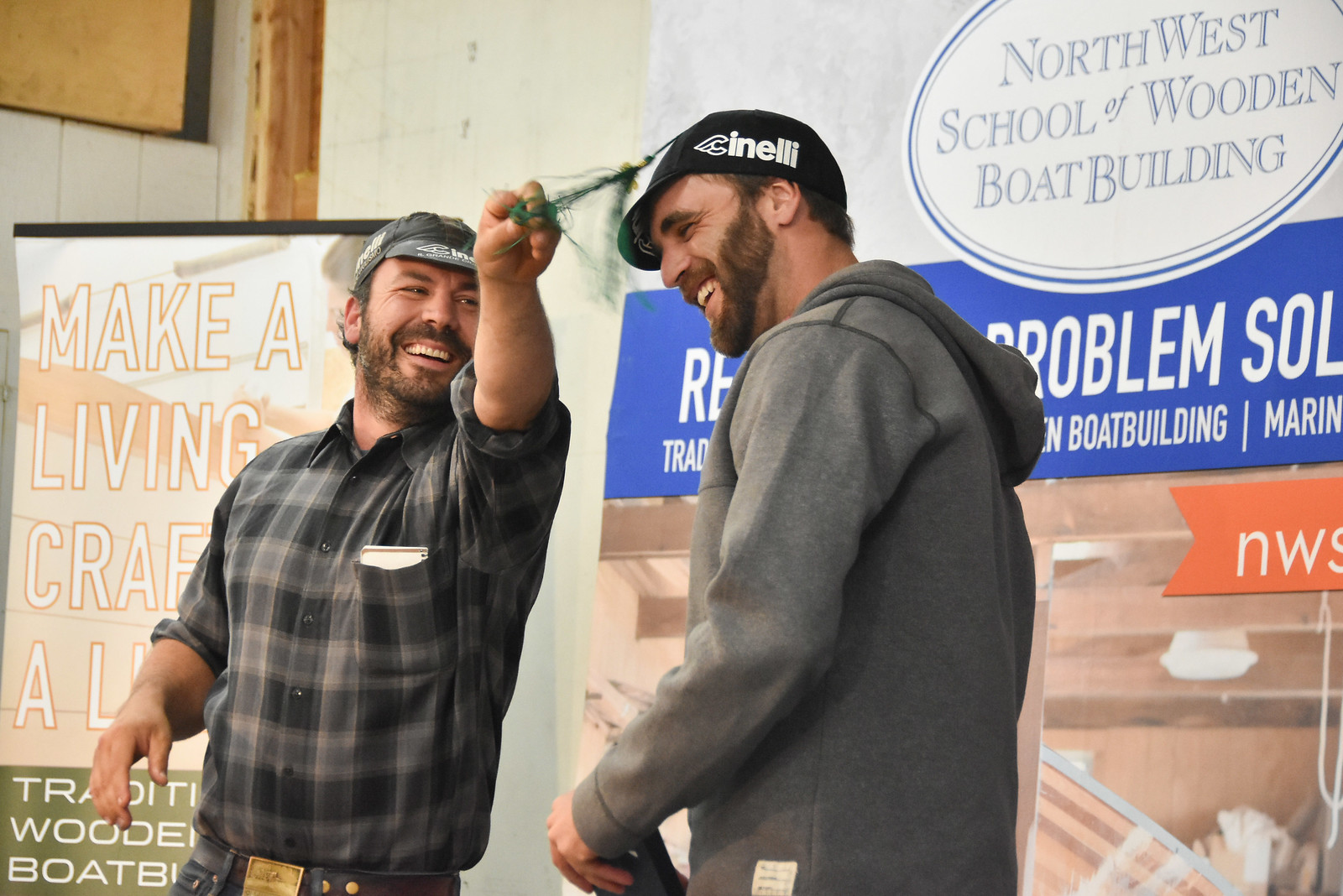The image depicts two Caucasian men from the waist up, seemingly caught in a moment of playful interaction and laughter. The man on the left sports a dark blue and gray plaid shirt with rolled-up sleeves, a gray hat, a beard, and denim pants. His shirt is buttoned up, and he appears to be pulling on a green tassel attached to the other man's black hat, which reads "Inelli." This man on the right, who has a beard and bushy eyebrows, is dressed in a gray jacket and hoodie. His head is tilted slightly downwards as he laughs. The background includes several advertisements. Prominently, there is a sign with a white, egg-shaped oval and blue outline that reads "Northwest School of Wooden Boat Building." Below this, a blue banner with white text partially reads "Problem Solved Boat Building" alongside a related image. Another visible advertisement states "Make a Living CRAFT," written in orange. The setting might be a stage, given the visibility and positioning of the signs. The background also features a white, possibly tiled wall. The overall feel of the image is one of camaraderie and light-heartedness amidst a setting focused on boat building.